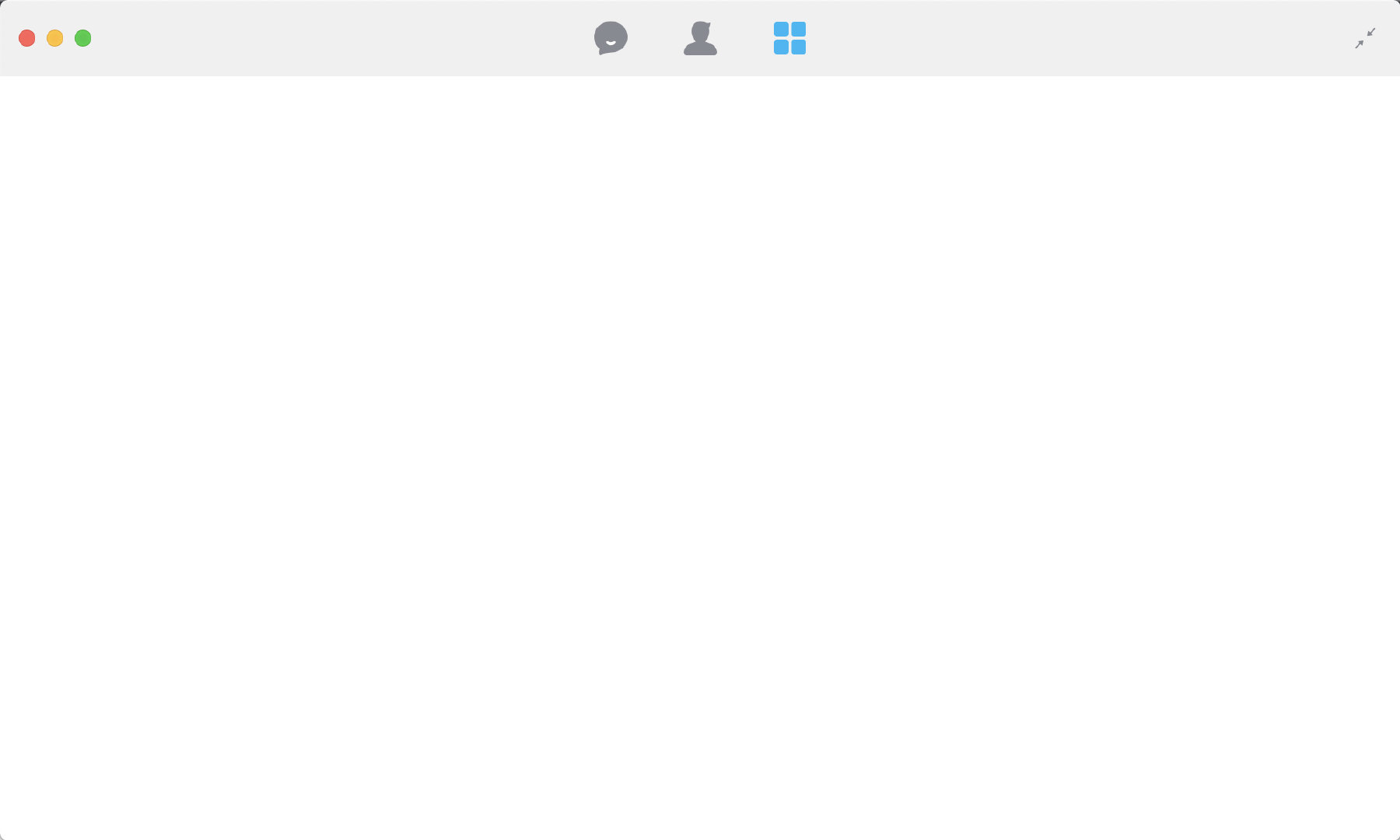The image appears to depict a digital whiteboard interface commonly used in virtual collaboration platforms such as Microsoft Teams or Zoom. Dominating the center of the image is a blank whiteboard space, prompting for input via drawing or writing. 

At the top of the interface, there is a gray toolbar containing three colored dots: a red dot for closing the whiteboard, a yellow dot for minimizing it, and a green dot for expanding it to full screen. 

Additionally, this toolbar features three icons: a thought bubble indicating a text or comment feature for user interaction, a silhouette representing the user's profile or participants in the session, and a set of four blue square-shaped boxes aligned in a grid, potentially symbolizing different tools or functionalities available on the whiteboard.

In the top-right corner, there is another minimize button. Overall, the interface is uncluttered, emphasizing simplicity and ease of collaboration.